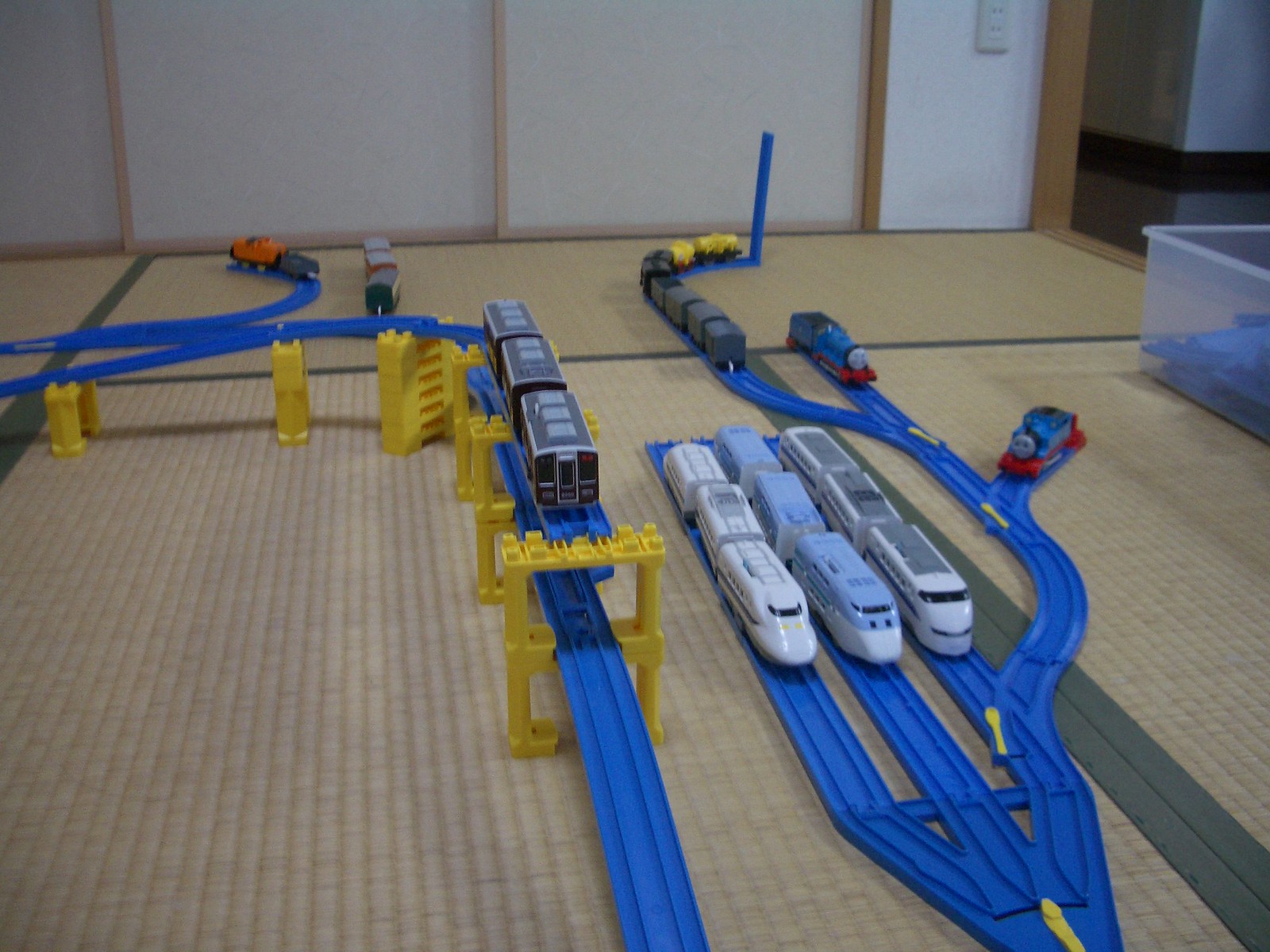This detailed photograph captures an elaborate toy model train set, meticulously arranged on a light-colored, possibly thatched or pile carpet floor. The train set features distinctive blue plastic tracks, including a section elevated by yellow pillars that transforms into a bridge. On the right side, three blue train tracks host a lineup of three parked commuter-like trains, each waiting at a makeshift station, with another train arriving from the back, accompanied by various carts.

A ramp on the left leads the tracks up and over the bridge, winding around with curves and eventually descending off-screen. Among the trains, there are notable appearances of Thomas the Tank Engine, along with other trains in colors such as gray, yellow, orange, light blue, white, and black. The scene is framed by white back walls and includes a clear storage tub holding additional track pieces, enhancing the realism and play possibilities of this engaging toy setup.